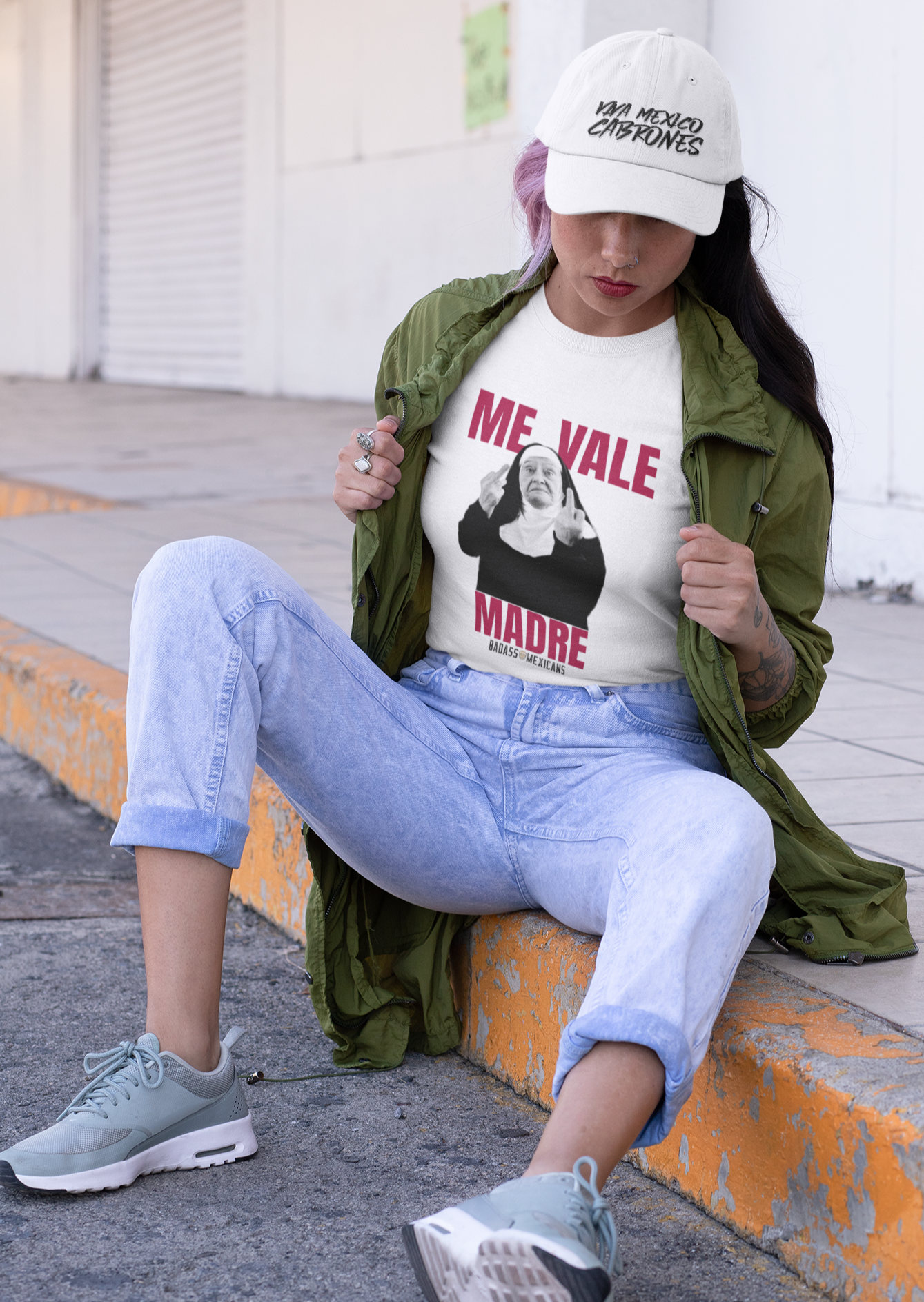A young Hispanic woman is sitting on a street curb during the daytime, seemingly posing for a photograph of her outfit. She has pink and black hair and is wearing red lipstick. She is dressed in light acid-wash denim jeans that are rolled up midway up her calves, gray and white sneakers, and an olive green, military-style jacket which she is holding open at her chest. Beneath the jacket, she is wearing a white t-shirt featuring a black-and-white graphic of a nun giving the middle finger with both hands. The shirt has red text reading "Me Vale Madre" with smaller black text beneath that says "Badass Mexicans." On her head, she sports a white baseball cap with the phrase "Viva Mexico Cabrones" in black lettering. She has tattoos on her left forearm and is wearing rings on her right fingers.